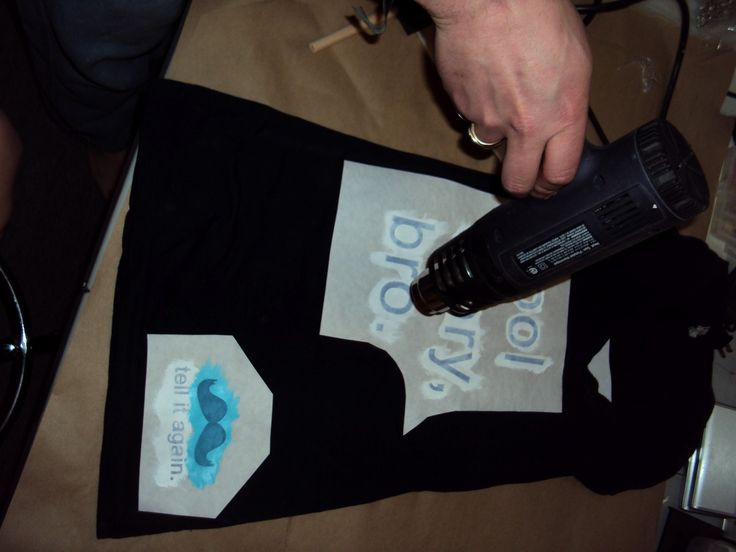In this image, a white hand with a ring on its ring finger is using a black industrial heat air gun to apply heat press images onto a black T-shirt. The T-shirt, which is laid out on a brown table, displays two sets of designs being transferred. The first design, positioned higher on the shirt, includes text that ends with the word "bro". The second design, located lower on the shirt's corner, features a drawing of a mustache with the words "tell it again" beneath it. The heat air gun, characterized by its trigger-like mechanism and an instructional safety label, is pointed directly at the lettering, which appears to be reversed as part of the transfer process. Surrounding the T-shirt are various objects, including what looks like an electronic device above the shirt and some arts-and-crafts materials to the left, indicating that the setting is likely a workspace or someone's home.